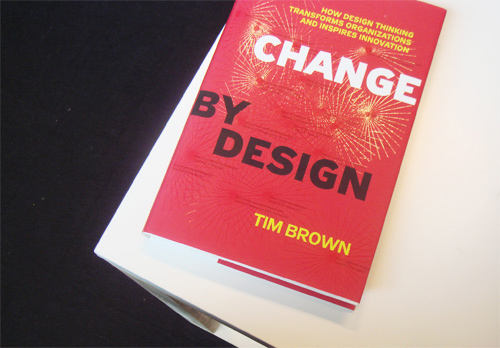The image is a top-down photograph of a book titled "Change by Design" by Tim Brown, placed on a white tabletop against a dark, barely discernible background. The book has a prominent red cover featuring a pale yellow, firework-like design behind the title, which appears to radiate outward like spidering bullet holes. The title "Change" is emblazoned in white font, while "By Design" is in bold black letters. At the top of the cover, in yellow font, are the words "How Design Thinking Transforms Organizations and Inspires Innovation." Similarly, the author's name, Tim Brown, is displayed in yellow at the bottom right corner of the cover.